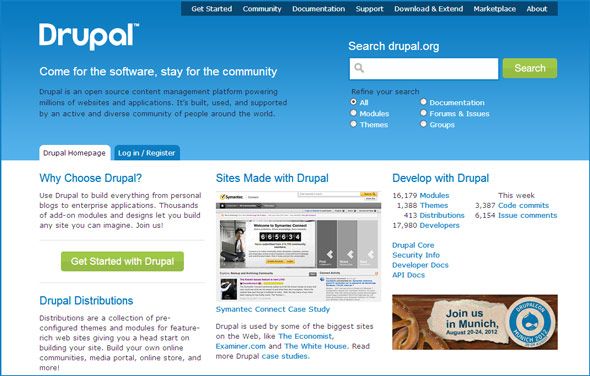The image depicts a segmented webpage from drupal.org. The rectangular image is divided into two sections: the upper half features a blue background, while the lower half is on a white background.

**Upper Section:**
- In the upper left corner, "Drupal" is written in bold white letters.
- Beneath it, in smaller white font, it reads, "Come for the software, stay for the community."
- In the center, a block of text in navy blue letters states: "Drupal is an open source content management platform powering millions of websites and applications. It's built, used, and supported by an active and diverse community of people around the world."
- To the right, in white letters, it says "Search drupal.org," with a search window below and a green button labeled "Search."
- Below the search bar, "Refine your search" is written in blue letters, followed by options such as "All," "Modules," "Themes," "Documentation," "Forums and Issues," and "Groups."

**Lower Section:**
- On the white background, a heading in blue letters reads, "Why Choose Drupal?"
- Below, in navy blue text, it says: "Use Drupal to build everything from personal blogs to enterprise applications. Thousands of add-on modules and designs let you build any site you can imagine. Join us!"
- Beneath this text, there’s a green bar with the words "Get started with Drupal" in white letters.
- The section continues with additional information and options spreading across the page.

The detailed segmentation and organized presentation of information guide the viewer through the features and benefits of using Drupal, emphasizing community support and versatility.